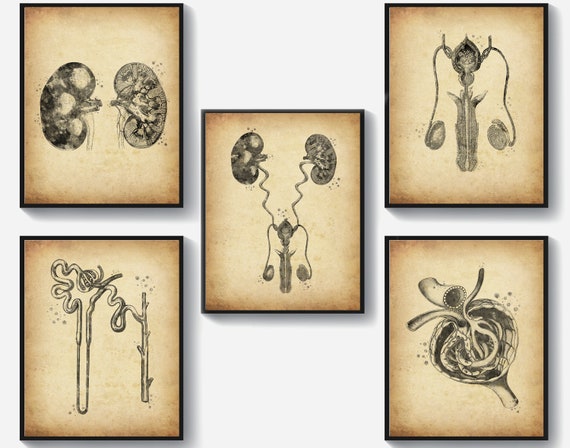The image consists of five detailed black and white anatomical illustrations, each encased in thin black frames against a background with a yellowish-brownish texture. The central drawing prominently features kidneys connected to what appears to be the urinary system. To the top left, there's a depiction of two kidney-like structures with distinct labels and markings, resembling Fallopian tubes or another part of the female reproductive system. The top right illustration shows an ovary filled with pink loops, attached to other structures via squiggly lines. The middle illustration portrays a cohesive view of these organs, possibly reflecting the entire female reproductive system, including the bladder. The bottom left corner contains a more abstract series of connected lines and shapes, possibly representing a detailed look into the internal pathways of these organs. Meanwhile, the bottom right image depicts a thick, orb-shaped tube extending upward, likely another component of the reproductive or urinary systems. Despite the detailed renderings, the absence of identifying text leaves the exact nature of some elements open to interpretation.